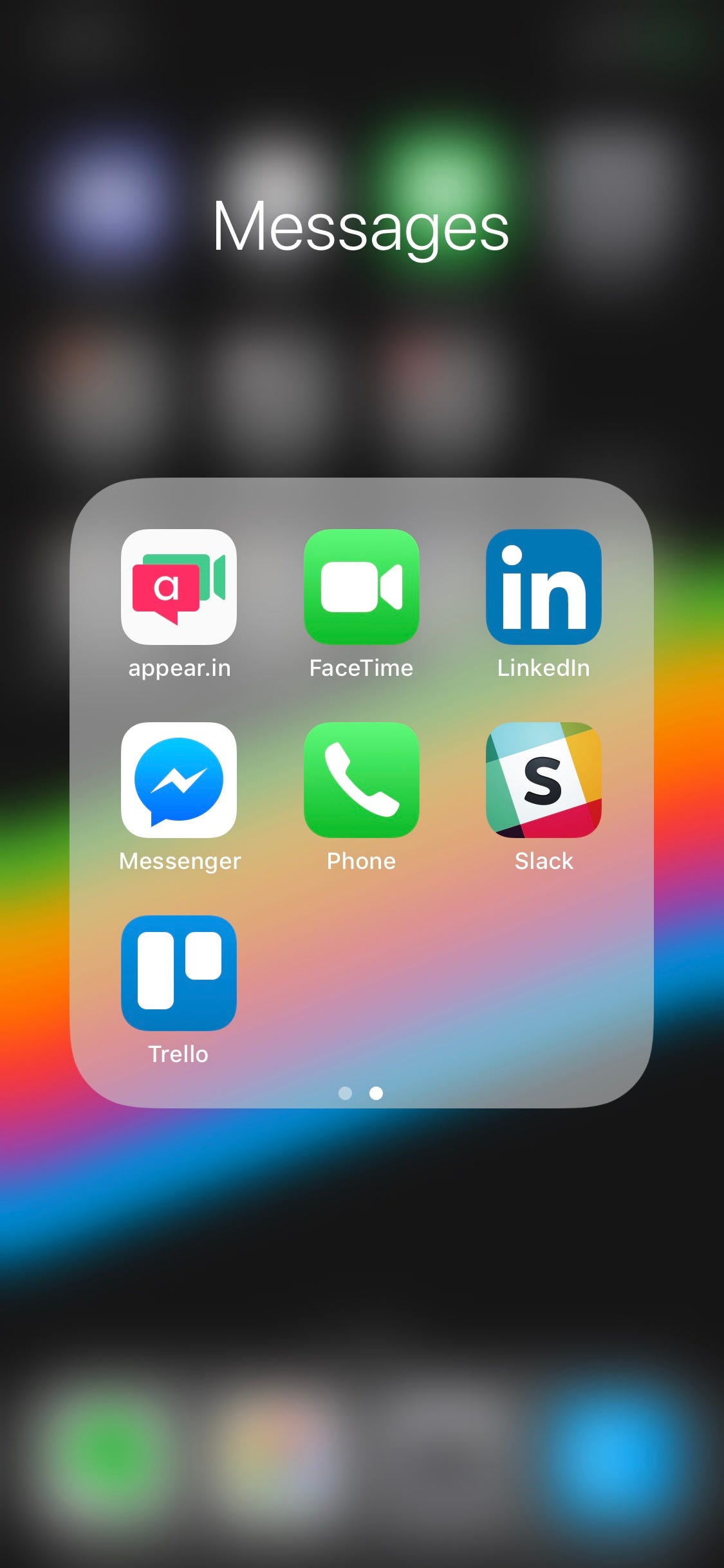This is a detailed screenshot taken from a smartphone, showcasing a vertically oriented, tall rectangular display. The background of the screenshot is predominantly blurred, featuring a gradient of colors including black, red, orange, purple, and blue. At the top of the screen, there are two lines of blurred icons, overlaid with the word "Messages" in a clear white font.

Central to the screenshot is a square, gray area with gently rounded corners. Within this square, three horizontal rows of icons are displayed. The first two rows each contain three icons, while the third row contains a single icon. The icons represent the following applications: Appear.in, FaceTime, LinkedIn, Messenger, Phone, Slack, and Trello. Each icon is clearly visible, set against the gray background, providing a concise view of the available communication and productivity tools on the device.